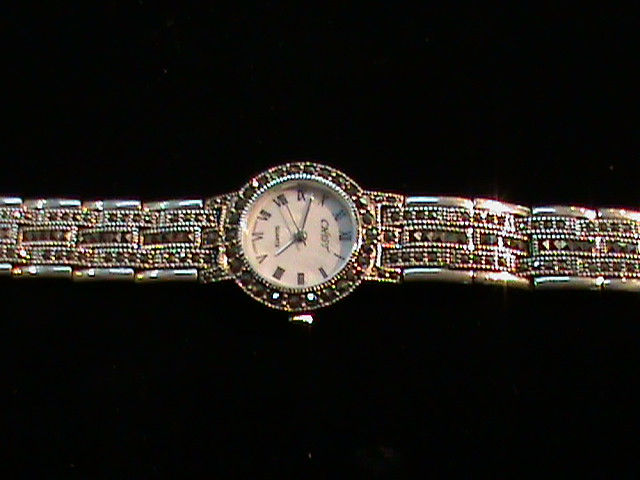The image captures a small, elegant, jewel-encrusted watch set against a solid black background. The face of the watch is predominantly white, adorned with simple Roman numerals and silver hour, minute, and second hands—the latter positioned around the 40-second mark, indicating the time as 4:47. The watch band, although only partially visible, exhibits a metallic and rhinestone or possible gemstone design, with hints of green likely suggesting emeralds. The brand name is somewhat blurred but appears to begin with a 'C' and end with a 'T', resembling names like Cabot or CADT, with the word "Corpse" faintly visible at the bottom. The watch incorporates a knob for winding on its right side and exudes a sophisticated aura suitable for formal evening events.